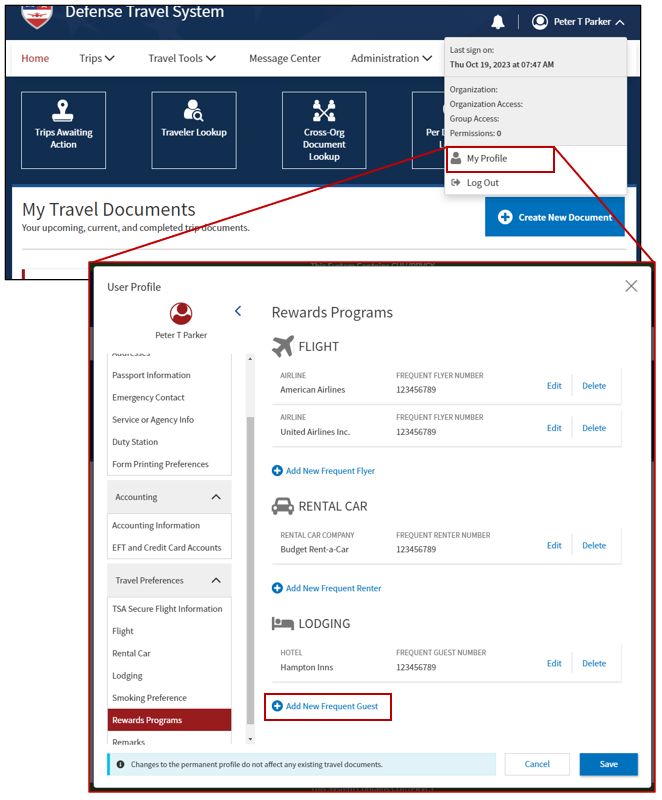This is a detailed vertical screenshot of a website accessible from a computer or smart device. The interface prominently features a dark blue banner across the top. On the upper left, there is an emblem next to the text "Defense Travel System." On the upper right, the banner includes a bell icon for notifications and a circular profile icon with the name "Peter T. Parker."

Below the banner is a white rectangular navigation bar. The 'Home' tab is highlighted in red, while other tabs—'Trips,' 'Travel Tools,' 'Message Center,' and 'Administration'—are in black. There is a pop-up box indicating the user's last sign-on was on Thursday, October 19th, 2023 at 7:47 a.m., along with organization and access details. The user's profile section features a red-bordered box with a logout button and lines extending to a user profile pop-up box.

Above, under the 'My Travel Documents' section, it details upcoming, current, and completed trip documents, with options to create new documents via a plus sign and a blue button. The dark blue background reappears above this section, showcasing several icons for functionalities like 'Trips Awaiting Action,' 'Traveler Lookup,' and 'Document Lookup,' among others, some partially obscured by a pop-up box.

The user's profile information, including Peter T. Parker’s details and reward programs for flights, rental cars, and lodging, is listed on the left-hand side. There are options to cancel or save information.